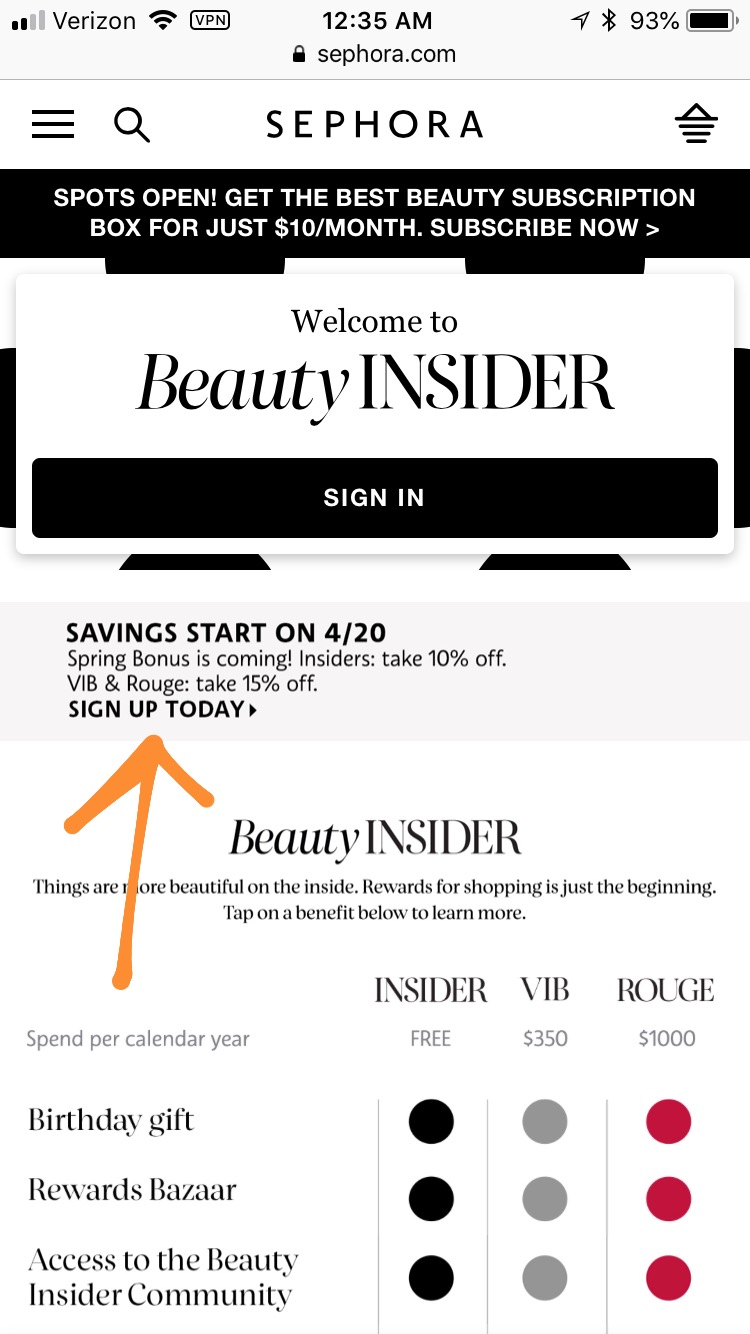This image is a rectangular, vertically-oriented screenshot, likely taken from a cell phone while browsing the Sephora website or app. The topmost section features a thin gray banner displaying typical cell phone status icons. On the top left, it shows a cell phone signal strength of 2 out of 4 bars and the network provider name, Verizon. Adjacent to this, a full-strength Wi-Fi signal icon is displayed, followed by a black-outlined box with the text "VPN" inside. Centrally, the time is displayed as 12:35 a.m. Below this, the URL "sephora.com" is indicated, and to the upper right, an arrow points diagonally upward. Next to this is a Bluetooth symbol accompanied by a "93%" battery icon, suggesting the battery is nearly full. 

A thin gray line separates this information from the next section, which features a white banner spanning the width of the image. On the left side of this banner is a hamburger menu icon composed of three horizontal lines, followed by a search icon. In the center, "Sephora" is prominently displayed. To the right, there is a triangle symbol at the top with diminishing horizontal lines beneath it.

Below this banner, a black box with white text promotes a beauty subscription box: "Spots Open - Get the Best Beauty Subscription Box for Just $10 a Month. Subscribe Now" with an arrow pointing to the right. Underneath, a white box welcomes users to Beauty Insider. This section is followed by another black box with white text that reads "Sign In."

[Please note that the content described is purely textual and visual details from an interface and does not depict actual products or detailed imagery beyond app informational icons and banners.]